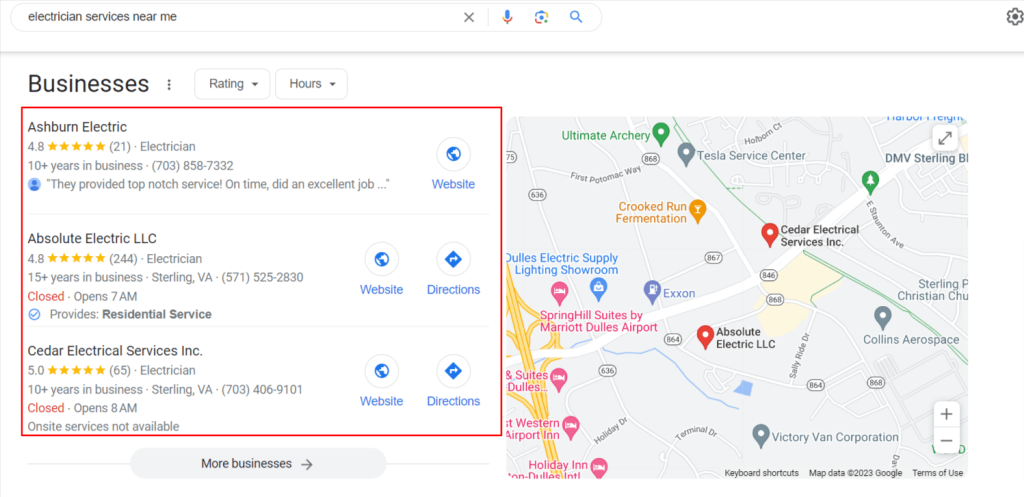Here's a detailed and cleaned-up caption for the image:

"The image showcases a double-pane layout featuring business listings and a corresponding map. In the top part of the image, there is a search toolbar reminiscent of the Google search bar, with options to input 'electrician services near me' and icons for voice search, image search, and a standard search.

Below the search bar, on the left side, is a column displaying business listings. Each listing includes the company name, rating, business type, contact information, and website link. The first listing is for 'Auburn Electric,' which has a 4.8-star rating. It indicates the business type as 'electrician' and provides both a phone number and a website link. 

The second listing features 'Absolute Electric, LLC,' also rated 4.8 stars, with details stating the business opens at 7 a.m. It includes a caption, phone number, website link, and a directions link.

The third listing is 'Cedar Electric Services Incorporated,' which boasts a 5.0-star rating. It highlights having '10 years in business,' provides a phone number, and mentions that the business opens at 8 a.m. Links to the website and directions are also provided.

Adjacent to these listings on the right is a Google map. The map marks each business location with red indicators for 'Absolute Electric' and 'Cedar Electric.' Additional points of interest, such as a fermentation plant marked with a yellow icon, and hotels including the Marion Hotel, Best Western, and Holiday Inn, suggest that the area is likely in a downtown city environment where these amenities are situated closely together."